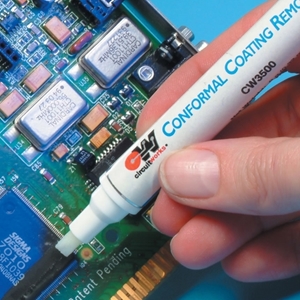The image shows a close-up of a person's hand holding a white-tipped marker from CircuitWorks, labeled "Conformal Coating Remover" with the model number CW3500. The person, who has a somewhat long thumbnail, is applying the marker to a motherboard, which features intricate circuits, green settings, wiring, and electronics. The motherboard section being worked on includes components marked "Sigma Designs 7010." This conformal coating remover appears designed to clean off any protective coatings on the motherboard, suggesting its use in electronics maintenance or repair work. The brand logo and product details are prominent, emphasizing the tool's specialized purpose.